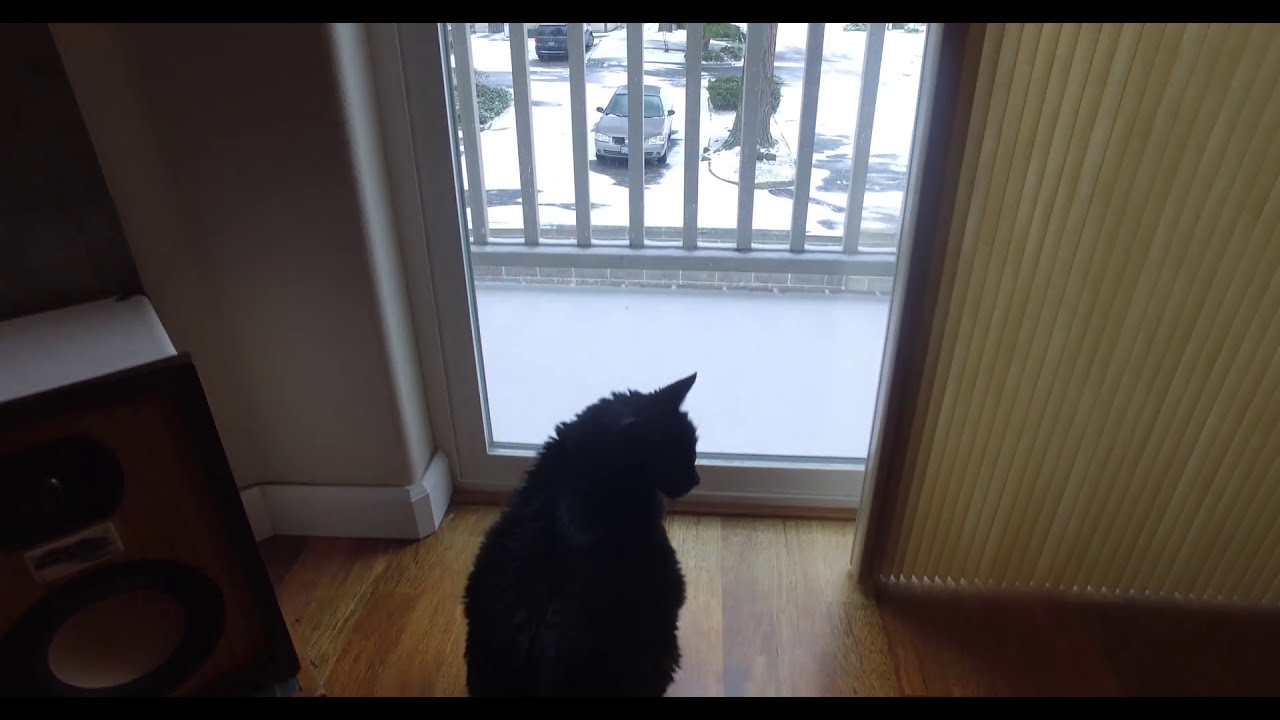The image features a wide rectangular shot of a cozy indoor setting with a black cat sitting on an orangish-brown wooden floor, gazing intently out of a glass door directly in front of it. The cat is positioned at the bottom of the image, presenting its silhouette with its back facing us, while its head is turned right, looking downwards towards the right corner. Notably, some fur stands out along its coat, giving it a textured appearance. 

To the cat's left is a speaker in a rectangular or cubic shape, characterized by wooden housing and two distinct white and black speaker areas. The left side of the image also reveals a light gray wall with white molding and a chair that appears to be black and white. 

At the center of the frame, the glass door has a white border and leads to an outdoor balcony paved with gray stones and safeguarded by a gray-colored metal gate. The balcony offers a view of a street below, where cars, including a silver and a black one, are parked amid several bushes and trees. The scene outside appears bright, suggesting it might be daytime. To the right of the cat, partially covering the door, are cream-colored blinds, adding a touch of warmth to the tranquil indoor atmosphere.